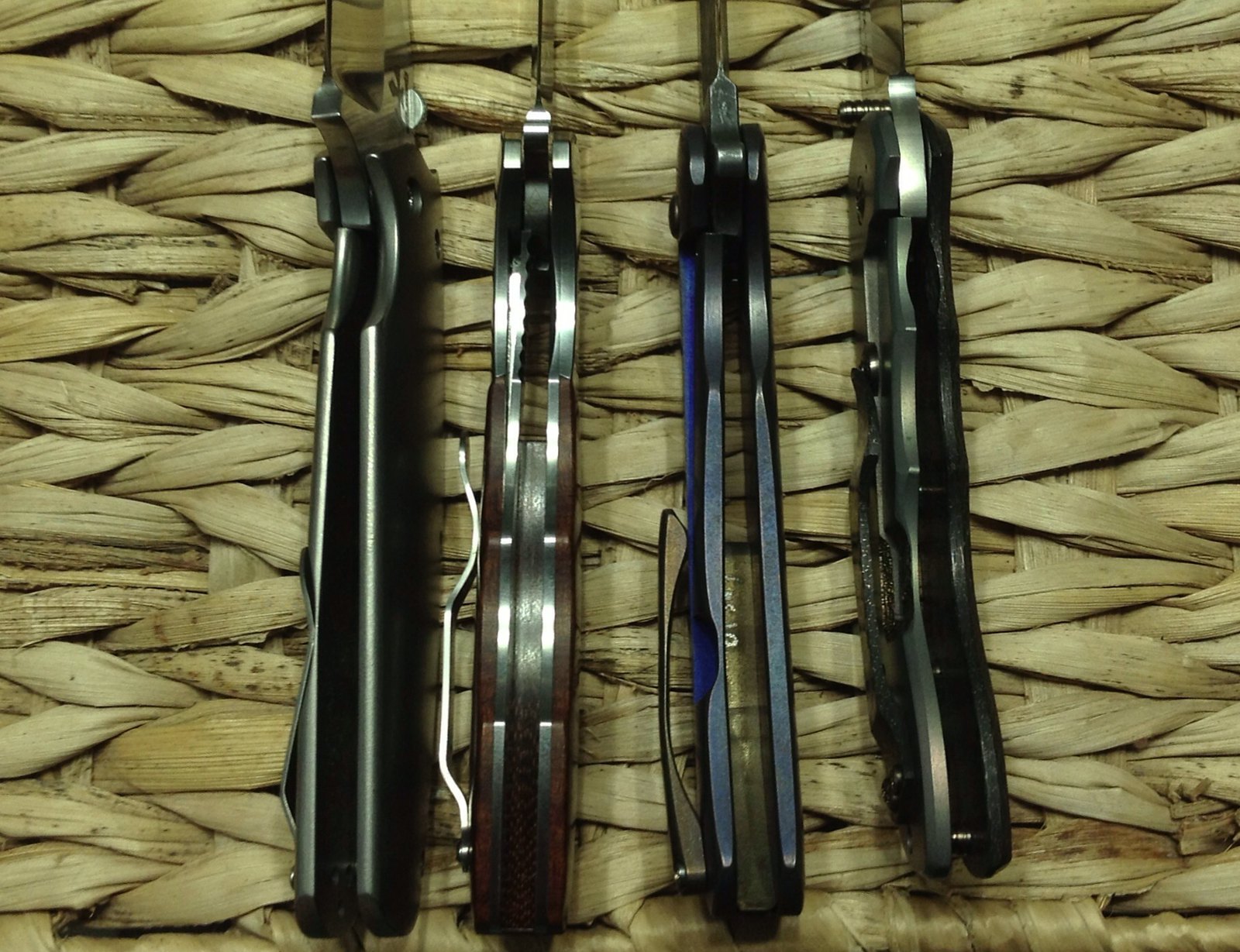This detailed photograph captures four modern pocket knives laid out on their spines with blades retracted, positioned upright on a tightly woven wicker or straw basket. Two of the knives feature sleek black handles, one exhibits a rich mahogany finish, and the fourth one is dark blue at the base. The knives' metallic components appear shiny and relatively new. Only the handles and a minor part of the blades are visible, revealing built-in clips designed for attachment to clothing. The positioning shows the thinnest part of their handles, giving a partial view of the folded area where the blades tuck in when not in use. Each knife possesses a unique quality, including a glitter design on one black handle, emphasizing their readiness, utility, and aesthetic appeal.